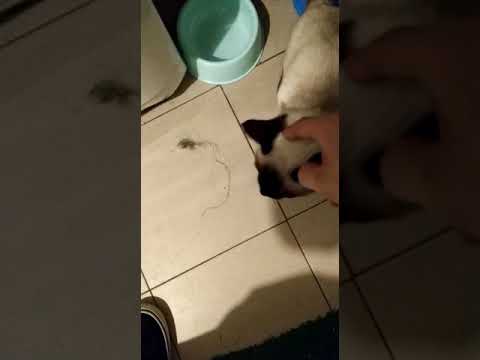In this image, we are looking at a screenshot or photo captured with a mobile phone, depicting a domestic scene on a tan tile floor, likely in a pet feeding area of a house. Dominating the upper right section of the image is a white and black cat, characterized by its black ears and markings around its nose. The cat is gazing towards the left side of the frame, while someone's hand, partially visible, gently pets the top of its head. Near the top center of the image, there's a small light blue water bowl. In the lower left corner, there is a blue shoe with a white sole, and in front of the cat, there's a small object that looks like either a toy mouse on a string or a tuft of fur. The image is framed by two semi-transparent black stripes on either side, slightly darkening the edges of the picture.